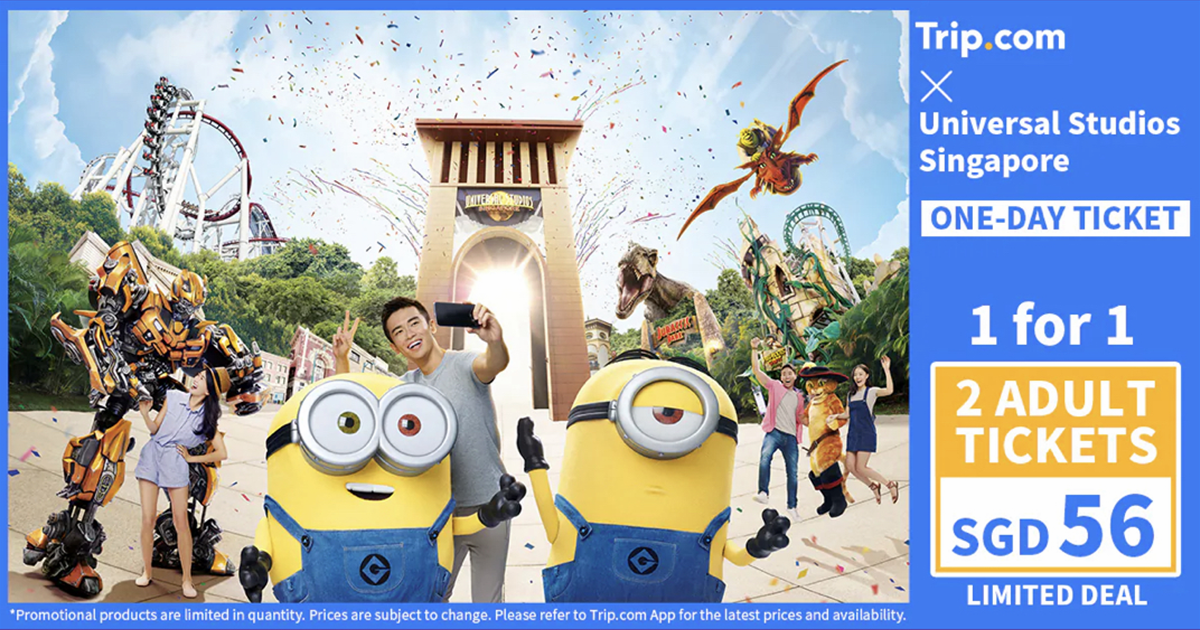This advertisement for Trip.com features a vibrant and detailed layout. The background is a rich medium blue color. Positioned on the right side of the ad, the top displays 'Trip.com' in white text, with a yellow dot. Below this, there's a white 'X' and the phrase 'Universal Studios Singapore' in white text. Further down, there's a white banner with the blue text 'One Day Ticket'. Beneath the banner, white text reads 'One for One', followed by another segment with a gold background. This section includes a squared box stating 'Two Adult Tickets' in white text, with its lower half on a white background displaying 'SGD 56' in blue text. Below this, in white text, it says 'Limited Deal'.

To the left of the text, a lively picture shows a group of Asians, approximately four or five people, taking a selfie. The focal point is a young man capturing the moment. In the backdrop, children are seen joyfully jumping, accompanied by Puss in Boots dressed up and standing between them. High above, a bird character can be spotted in the sky. The background is busy with a dinosaur, and to the left side, a roller coaster looms. Additionally, a girl at the bottom left is seen posing in front of a Transformer, adding to the fun-filled ambiance of the image.